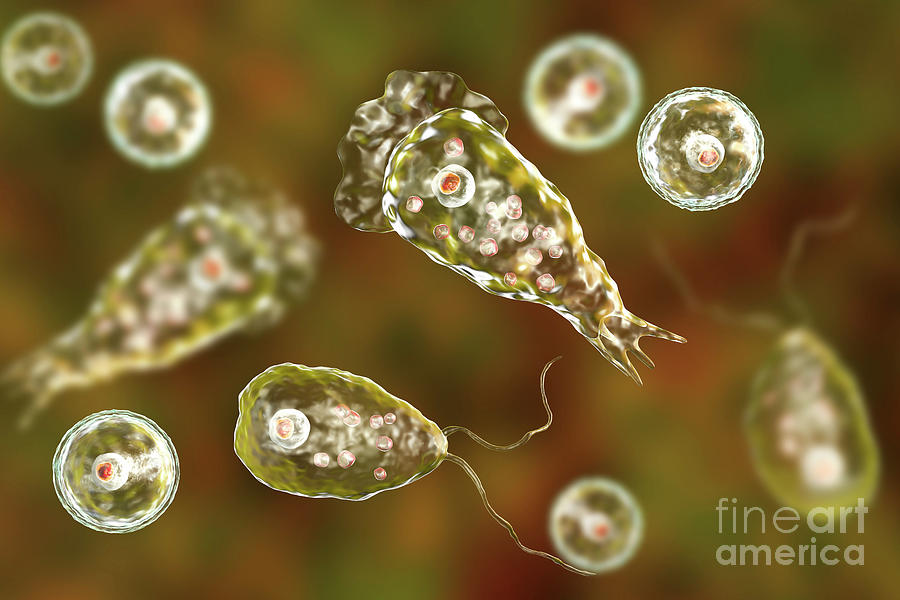This digitally rendered image, reminiscent of something seen under a microscope, vividly captures single-celled or very few-celled translucent organisms. Each organism is portrayed in meticulous detail, with one prominent in the center, featuring red dots and bubbles inside. Surrounding this central figure are both tubular and circular shapes, some with additional features like tendrils or antennae. The organisms exhibit a variety of colors, specifically pink, yellow, green, and white, standing out against a blurred pink, green, and brown background. There are four organisms prominently displayed in the foreground, with six more faintly visible in the blurred background. In the bottom right-hand corner, the image is discreetly marked with "Fine Art America," adding a touch of authenticity to this artistic representation of microscopic life forms.